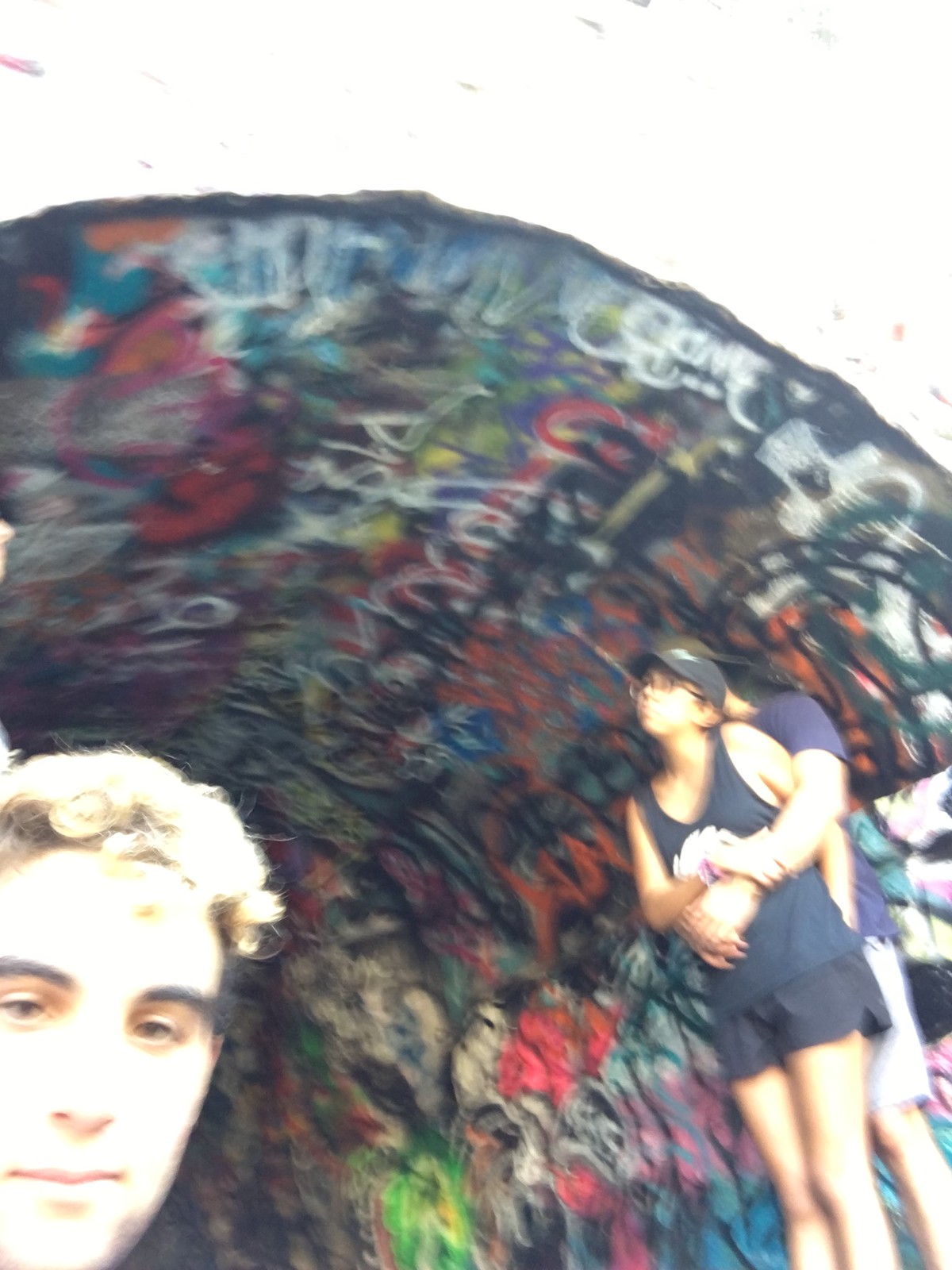In the photograph, we observe three individuals partially visible. They are situated at the entrance of a heavily graffiti-covered tunnel. The graffiti, a chaotic blend of red, white, black, green, and blue hues, layers the upper sections, making it difficult to discern specific details due to the lighting conditions.

On the right side of the image, a couple stands in an intimate pose. The man, whose face is obscured as he stands behind the woman, is dressed in a black shirt and gray shorts. His arms are wrapped around the woman, whose appearance is more clearly captured. She dons a black hat, black tank top, black shorts, and glasses, and is seen holding the man’s arms while looking upwards.

To the left, in the corner of the frame, only the partially obscured face of another male is visible. He has distinctive black eyebrows and blonde hair, though evidence of natural dark roots suggests his hair is dyed.